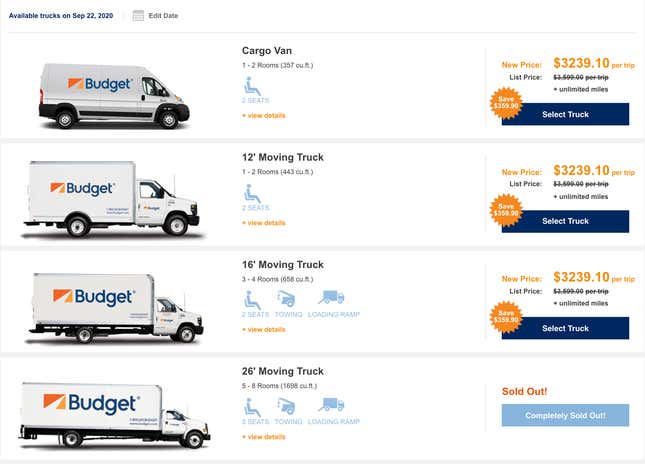**Detailed Descriptive Caption:**

The image is a screenshot displaying various budget van options available for rental, dated September 22, 2020, as indicated by small blue lettering in the top left corner beside a calendar icon and edit date option. The primary content is organized into labeled sections.

At the top of the listing is a cargo van, identifiable by the "Budget" branding on its side. This van is described as suitable for moving one to two rooms and has two seats. The associated benefit of "review details" is highlighted. To the right, pricing and information are clearly presented: the new rental price is listed as $3,239.10 per trip, a previous list price is crossed out, and the offer includes unlimited miles with a noted saving of $359.90. The rental option concludes with a "Select Truck" button.

Below the cargo van is a 12-foot moving truck, featuring a semi-truck design but shorter in length. This vehicle, also fit for moving one to two rooms and equipped with two seats, shares the same pricing structure—$3,239.10 per trip with a savings of $359.90—and an identical "Select Truck" button.

Further down, a 16-foot moving truck is presented. This larger option is able to accommodate three to four rooms and includes additional features such as towing capabilities and a loading ramp. Once again, the price stands at $3,239.10 per trip, with the same savings of $359.90 advertised.

Finally, the longest vehicle in the listing is a 26-foot moving truck, suitable for moving five to eight rooms. This truck also features towing capabilities and a loading ramp. It emphasizes its status, displaying "Sold Out" prominently, with the accompanying button marked as "Completely Sold Out."

Overall, this comprehensive screenshot offers a detailed view of available budget van options, complete with specifications, pricing details, and status indications for each vehicle type.